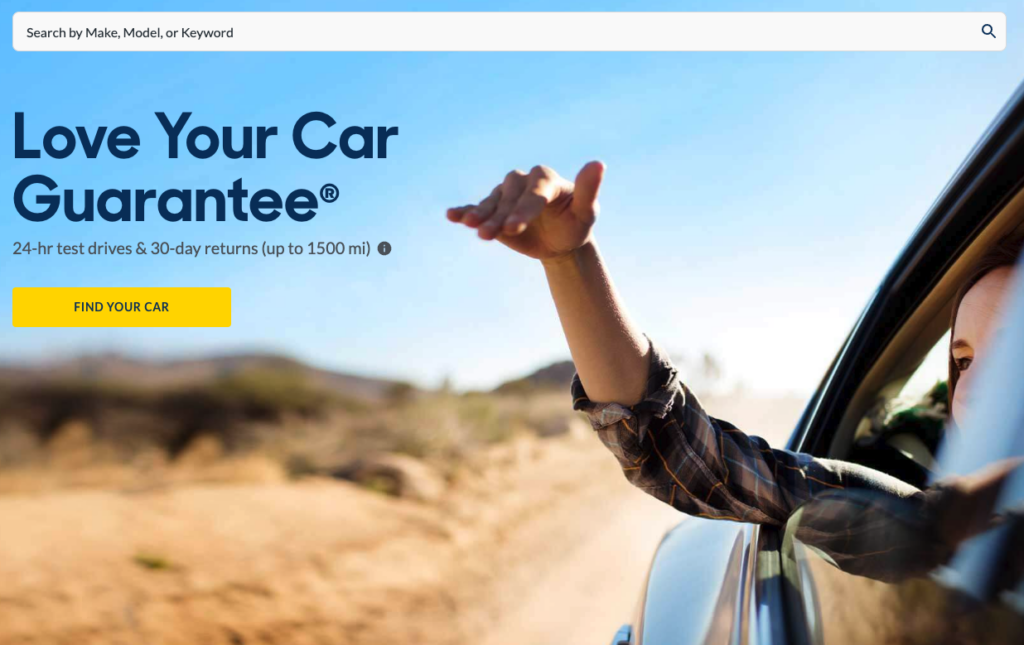In this image, we see a daytime desert-like landscape captured in a screenshot. Prominently on the right side, there's a partial view of a dark-colored car, with the window rolled down. A young woman with fair skin and dark hair is partially visible, showing her right eye, part of her profile, and her right arm resting on the window's edge. She is wearing a long-sleeve plaid shirt with the sleeve neatly folded up. The desert terrain outside features sandy ground interspersed with blurred low-lying greenery. Distantly on the far left, a small mountain range is discernible against a clear blue sky. In the upper left corner of the image, bold text reads "Love Your Car Guarantee," with smaller text below stating "24-hour test drives and 30-day returns." The car surface reflects the surrounding environment, adding to the scene's expansive desert feel.